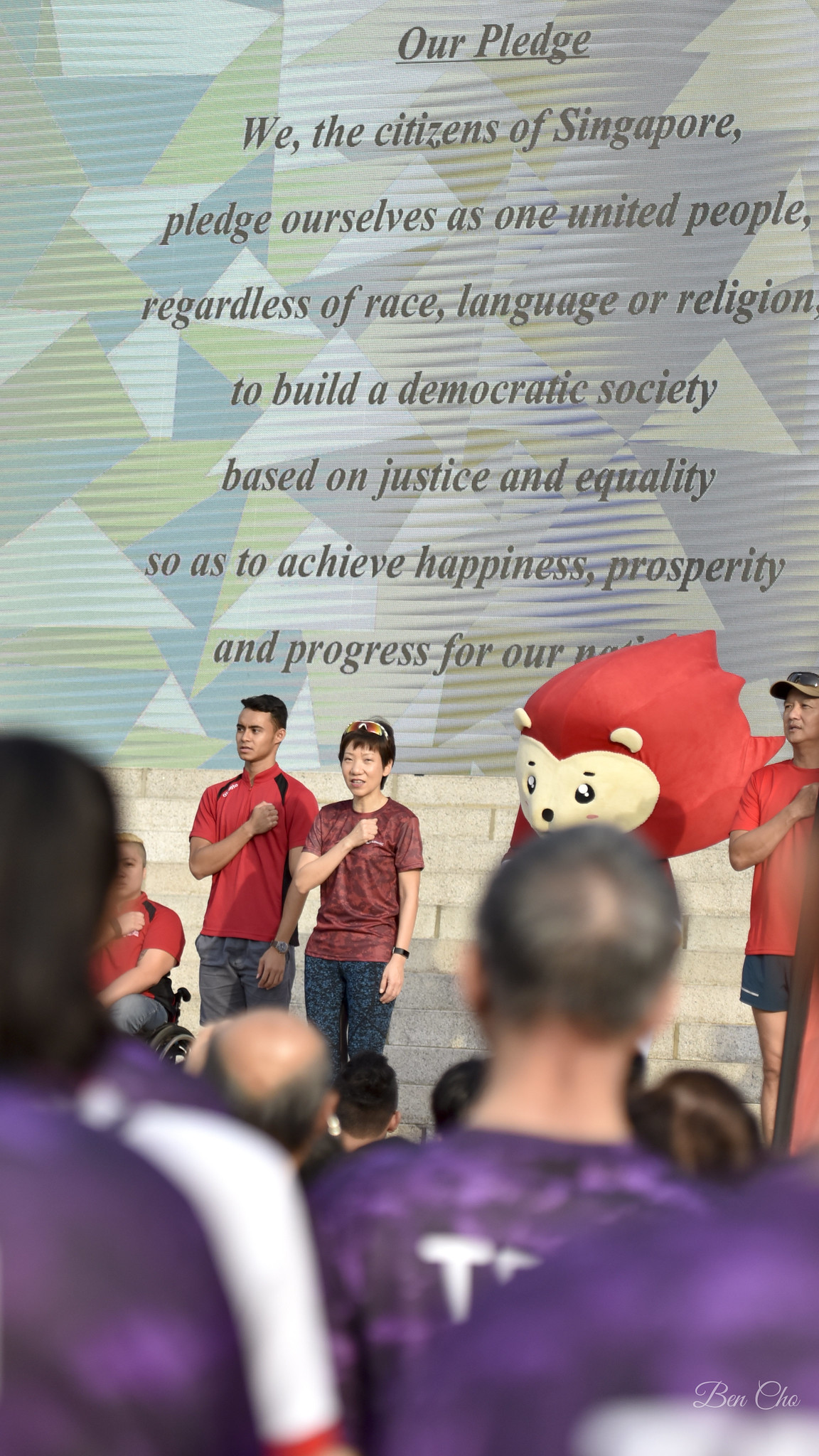In this photograph, the scene captures a patriotic moment where three individuals are standing at the forefront, their right hands placed over their chests in a pledge. They appear to be reciting the Singapore National Pledge, as visible text reads, "Our pledge, we the citizens of Singapore, pledge ourselves as one united people regardless of race, language or religion to build a democratic society based on justice and equality so as to achieve happiness, prosperity and progress for our [nation]." Although a part of the text is obscured, the commitment to national unity and progress is clear.

The three people in the front are joined by a mascot with red hair, resembling a chipmunk, adding a touch of charm to the scene. To the left, partly blocked from view, is an individual in a wheelchair. All three prominent figures are dressed in red shirts paired with black jeans or shorts, symbolizing unity and perhaps a shared purpose or team.

The audience, primarily dressed in purple shirts, is attentively facing the pledgers, creating a sea of purple that shows their unified presence and support. The background is a mix of vibrant energies and the solemnity of the pledge, depicting a moment of national pride and collective aspiration.